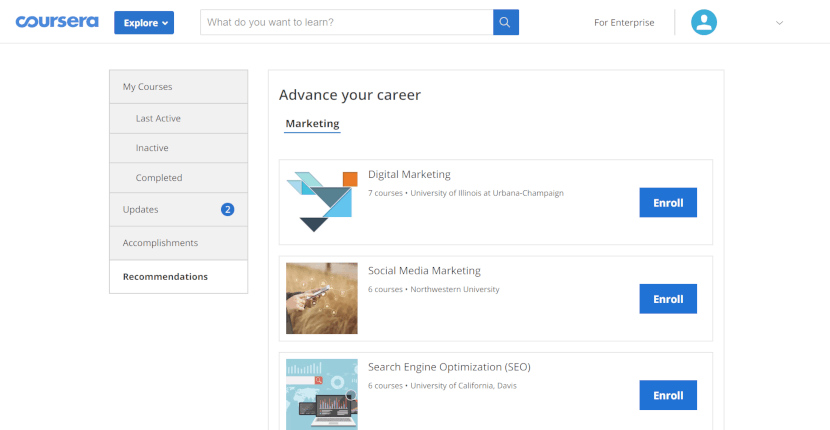This is a cropped screenshot of the Coursera online learning website, showcasing its clean and user-friendly interface. 

In the top left corner, the Coursera logo is prominently displayed. To its right, there's a drop-down menu labeled "Explore". Adjacent to this menu is a large search box with placeholder text in small grey letters reading "What do you want to learn?". On the far right, there's a link labeled "For Enterprise" in small grey letters. Beside it, a blue circle with a white profile icon indicates the user profile area.

Below this header section, to the left, a small vertical sidebar lists various options. The first section, labeled "My Courses", categorizes courses into "Active", "Inactive", and "Completed". The second category, "Updates", has a blue notification circle with the number "2". Following this, sections for "Accomplishments" and "Recommendations" are listed, with "Recommendations" being selected and highlighted in white.

To the right of the sidebar, a large central box encompasses the main content. At the top left of this box, the header "Advance Your Career" is followed by the subheader "Marketing" in small black letters. Below this, a vertical list displays three courses, each following a uniform format. The first course, "Digital Marketing," indicates it includes 7 courses and is hosted by a university. To the right of this course listing is a square "Enroll" button. The subsequent course listings follow the same structure, featuring thumbnails on the left, course titles to the right, additional course information beneath the titles, and "Enroll" buttons on the far right.